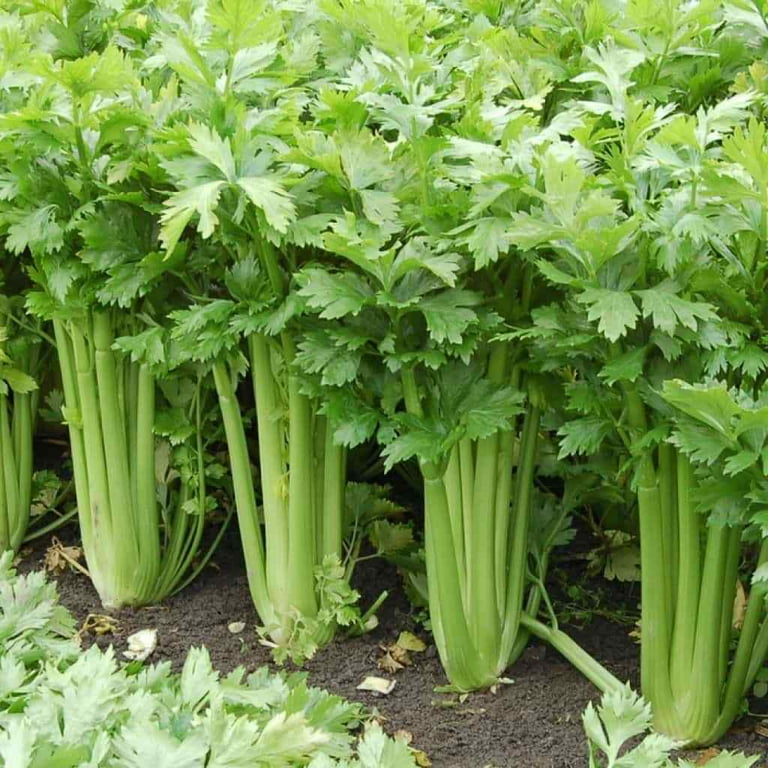The image captures a somewhat close-up view of a dense row of healthy celery plants growing in rich, dark brown soil. The scene is bathed in natural sunlight, although the sky is not visible. Each celery stalk, which consists of a lighter green hue transitioning to white at the base, stands upright, resembling miniature trees similar to broccoli. The sturdy stalks are crowned with a lush canopy of medium dark green leaves that fan out in overlapping layers, creating an impression of a verdant, leafy cover. In the foreground, at least four full celery stalks are prominently visible, with a few more partially seen toward the left. Scattered around the ground are random pieces of dead leaves, adding a natural, rustic touch to the vibrant setting. The entire patch of celery plants looks extremely healthy, mirroring the familiar form seen in grocery stores but rooted firmly in their natural growing environment.